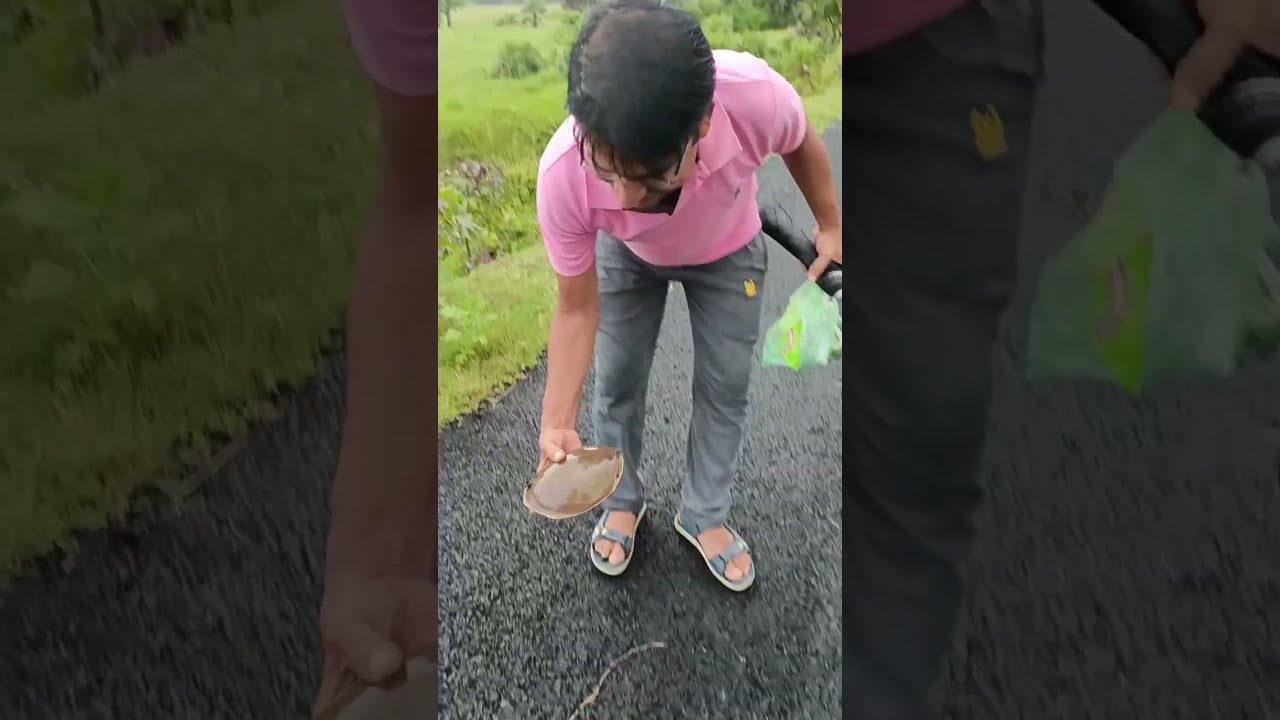In this vertical cell phone snapshot, a man is captured standing on a coarse, dark asphalt pavement pathway. The backdrop features an enlarged, faded version of the same scene, centered on the image. The man, dressed in a pink polo shirt, gray pants, and gray-strapped sandals, is slightly bent forward as he attentively examines a turtle in his right hand. The white man with black hair and glasses appears to be helping the turtle, potentially to cross the path. The turtle's smooth, brown shell glistens, indicating it might be wet, and its limbs are retracted inside. Behind the man lies a lush, grassy field filled with vibrant green shrubbery. His left hand holds what seems to be a green Swiffer and possibly a mic, adding to the curiosity of the scene.